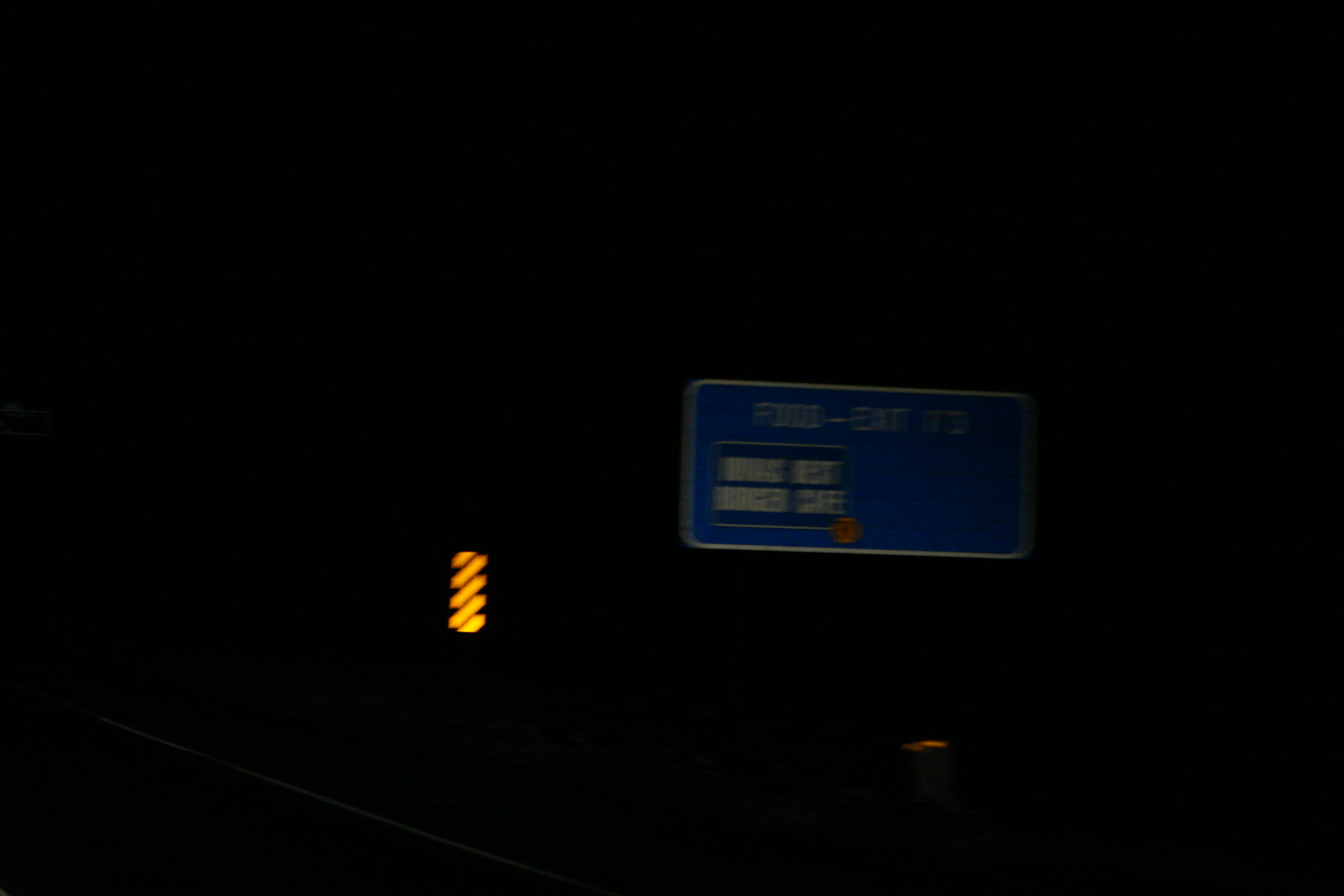This is a color photograph taken at night, likely from a moving car, given its extreme darkness and blurriness. Most of the image is pitch black, with only a few distinguishable elements. In the center, there is a glowing, reflective yellow sign with black diagonal stripes, indicating a bend in the road. To the right of this sign is a blue and white highway sign, partially readable with the word "exit" and the number "173". The exact establishment listed on the sign is illegible due to the blur. A faint white fog line is barely visible along the edge of the road. There are no discernible people, animals, buildings, plants, or vehicles in this photograph.